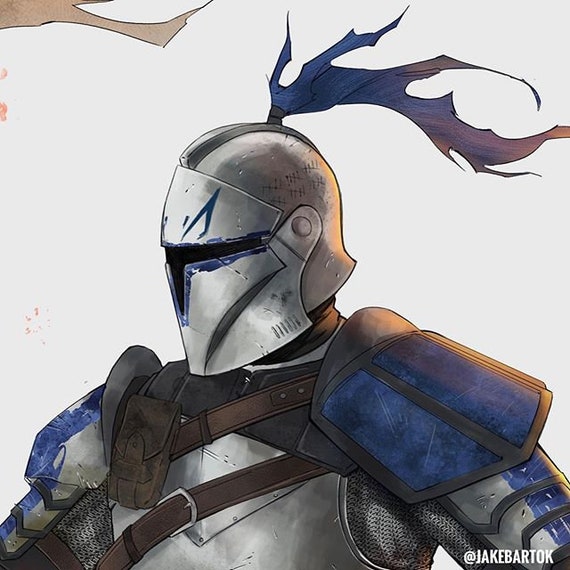This image is a detailed, color illustration of a medieval fantasy knight, formatted in a square. The background is a light gray, with a hint of a light brown tree limb in the top left corner. The knight, depicted from the top of the helmet to about mid-chest, is facing slightly toward the left. The armor is a mix of silver and blue, with blue shoulder plates and decorative blue markings. The helmet features a visor on the bottom portion, a black slit in the middle, and a striking dark blue plume that transitions to brown. Leather straps cross the knight's chest over chainmail under-armor. Notably, the helmet displays tally marks, possibly indicating 30 confirmed foes. The image is signed with white text in the bottom right corner reading "@Jake Bartok," indicating the artist.